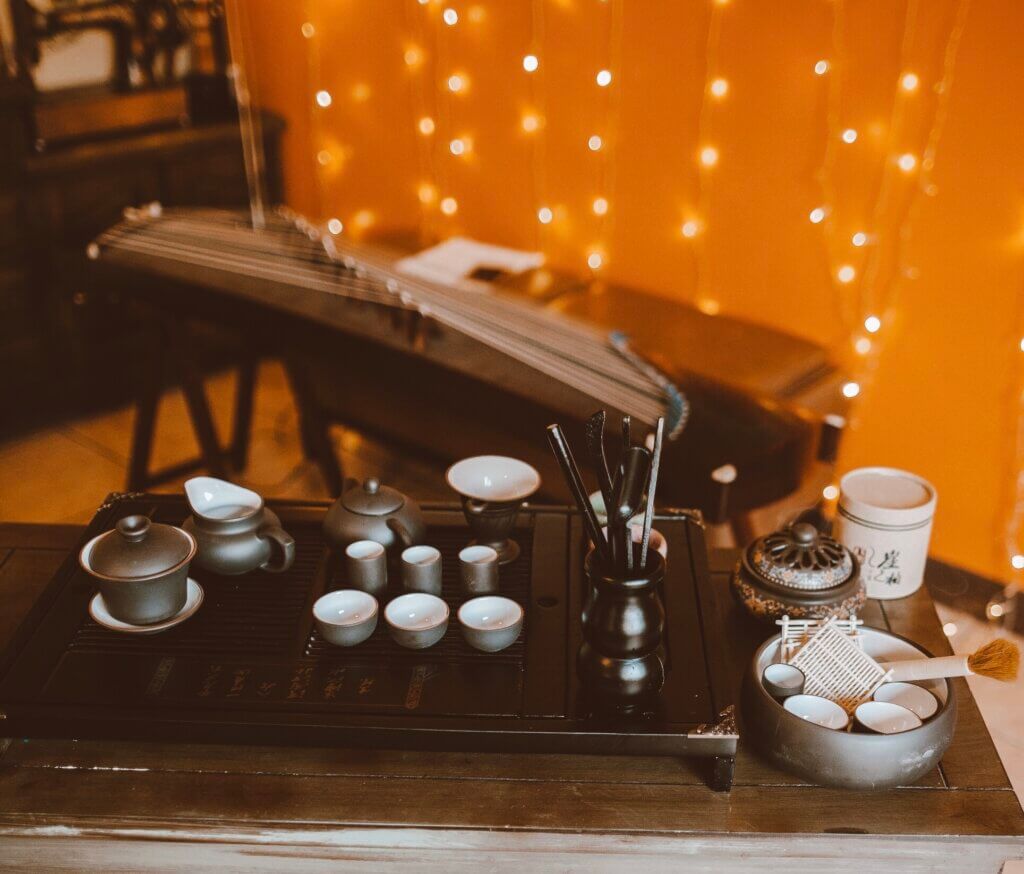This image showcases a detailed setup on a wooden table, positioned against an orange-colored wall adorned with twinkling string lights. At the center of the scene is an ornate wooden tray, which serves as the focal point, containing a variety of items. The tray holds several pewter cups and saucers, including a couple of larger mugs and much smaller bowls or Demitassi cups. One of the cups on the left side has a lid. Among these are also a sugar bowl and creamer, all finely organized.

To the right on a secondary tray, there is an assortment of other small circular dishes, possibly for tea or condiments, along with what seems to be a tiny stove or raised hot plate. Positioned on this are more pewter items, potentially makeup brushes or utensils, held in a small vase. This vase shares space with a container filled with what appear to be pencils or pens.

In the background, slightly blurred but adding to the ambiance, is either a shelving unit or a bookshelf made of dark wood that harmonizes with the wooden elements in the forefront. The overall lighting and intricate arrangement of containers, dishes, and utensils create a warm and welcoming vignette.